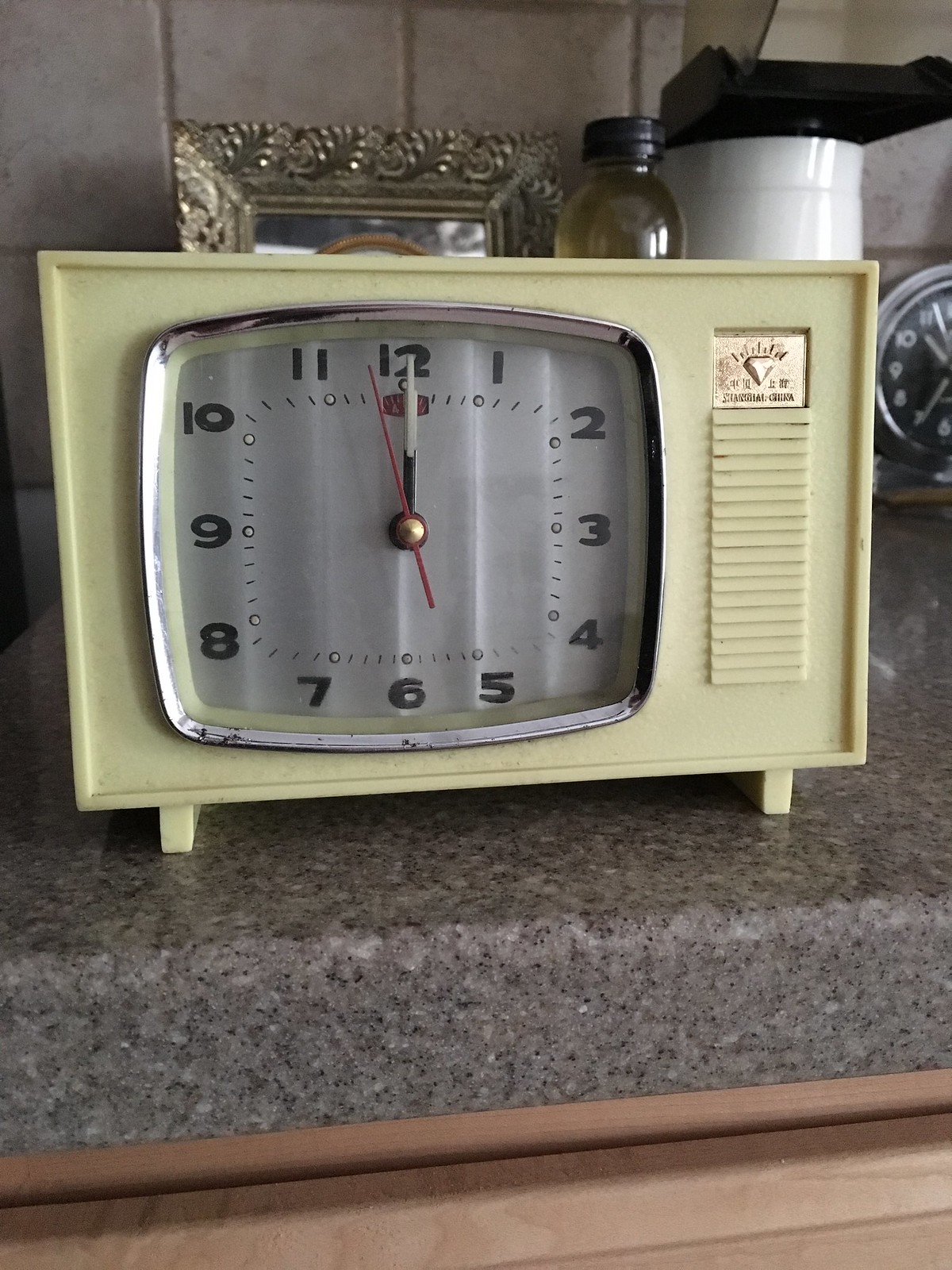This photograph captures a quaint and stylish marble-topped table, possibly a nightstand or a kitchen sink, with a surface of speckled white, grey, and black stone. Beneath the countertop, there are light brown wood drawers and cabinetry. Central to the composition is a vintage-style clock designed to resemble an old-fashioned TV. The clock has a pastel green, boxy frame with a rounded silver rectangle in the lower left. The main face of the clock is white-grey with black numerals from 1 to 12, and its hands are black and white with a red second hand, set precisely at a couple of seconds before 12 o'clock midnight. On the right side of the clock, there is a vent and a gold rectangle-shaped emblem with a diamond pattern and text reading "Shanghai, China." The overall design is reminiscent of the bulky, blocky style of old televisions or microwaves, complete with four legs. Behind the clock, there are pictures, a tea maker or water dispenser, a bottle of tea, and another clock, contributing to the old-world charm of the setup.